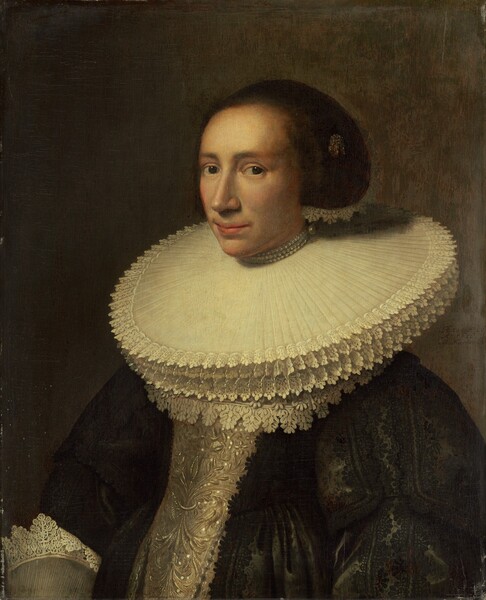This is a highly detailed portrait painting of a woman, possibly from the Victorian era, situated against a dark brown background. The woman, who is white, is adorned with a modest amount of makeup and exhibits a very subdued, closed-mouth smile. Her brown hair is styled in an elaborate updo, reminiscent of a quiffed snail shape.

A striking and grand adornment encircles her neck, resembling a giant frilled platter. It is meticulously pleated and crimped, with visible lace extending out to cover her shoulders. She wears a large, greenish-black robe, complemented by an ornate, decorative material or jewel-adorned silk descending the center of her body.

Her right wrist is visible, encircled by delicate lace. The attire also includes a black jacket with white lace at the collar and sleeves. Adding to her noble appearance, she wears a silver necklace, and her gaze is directed thoughtfully to the left. The painting's intricate details reflect a sense of opulence and historical elegance.